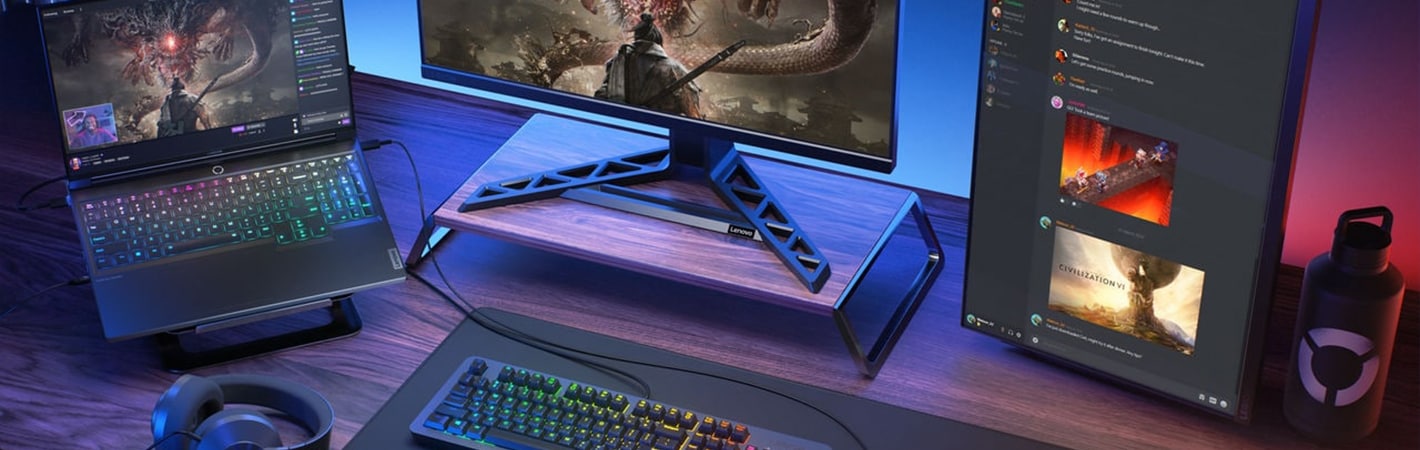The image depicts a meticulously arranged gaming and streaming setup on a dark brown wooden desk. Prominently in the bottom left corner, a pair of headphones rest on the desk. To the right of the headphones, a large mousepad supports a brightly lit, rainbow-colored keyboard. Above this, a laptop on a stand also displays a rainbow-lit keyboard and is running what appears to be a game resembling Elden Ring or Dark Souls, likely being live-streamed on Twitch.

To the right of the laptop, a monitor elevated on a wooden stand shows the same game without the streaming interface. Further to the right, a vertically oriented screen displays a Discord server with readable pictures and text. A black water bottle with a silver logo is situated at the far right end of the desk, adjacent to the vertical monitor. The entire setup suggests a professional gaming and streaming workstation, featuring vibrant RGB lighting and sleek peripheral organization.